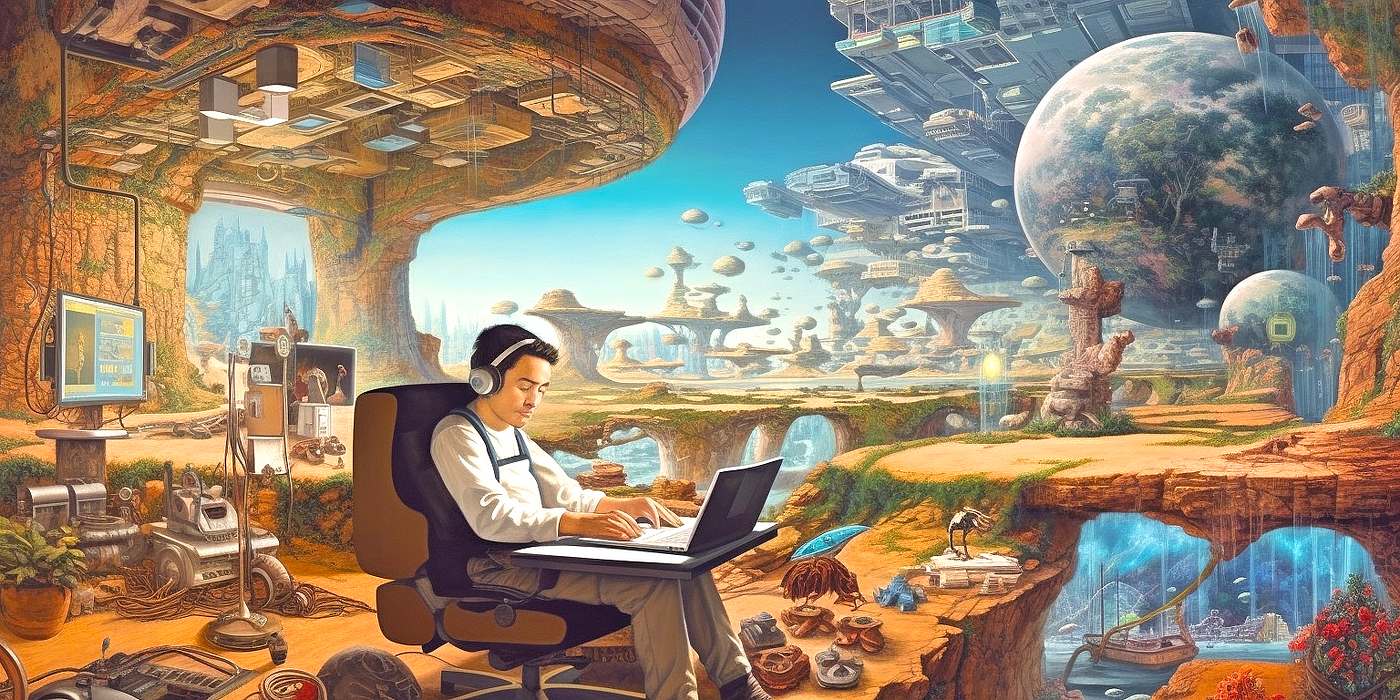This detailed, wide, landscape-oriented artwork features a young man with dark hair and white skin, wearing a white long-sleeve shirt and khaki pants, seated in a black gaming chair. He is engrossed in typing on a laptop that rests on a flip-up lap desk attached to the chair, while he wears headphones and looks down at the keyboard with closed eyes. The background is an intricate and otherworldly scene, depicting a futuristic, rocky, and botanical landscape resembling a sci-fi desert planet. To the left, a large, dirt-like awning supports an upside-down city, and several small robots and electrical equipment are visible. To the right, an Earth-like orb with a city peeking out from behind it floats at the top, with a lake beneath and water cascading down. The bottom right corner hosts a large boat beneath a cave, adding to the surreal and complex setting that envelops the focused individual amidst an emerging civilization.